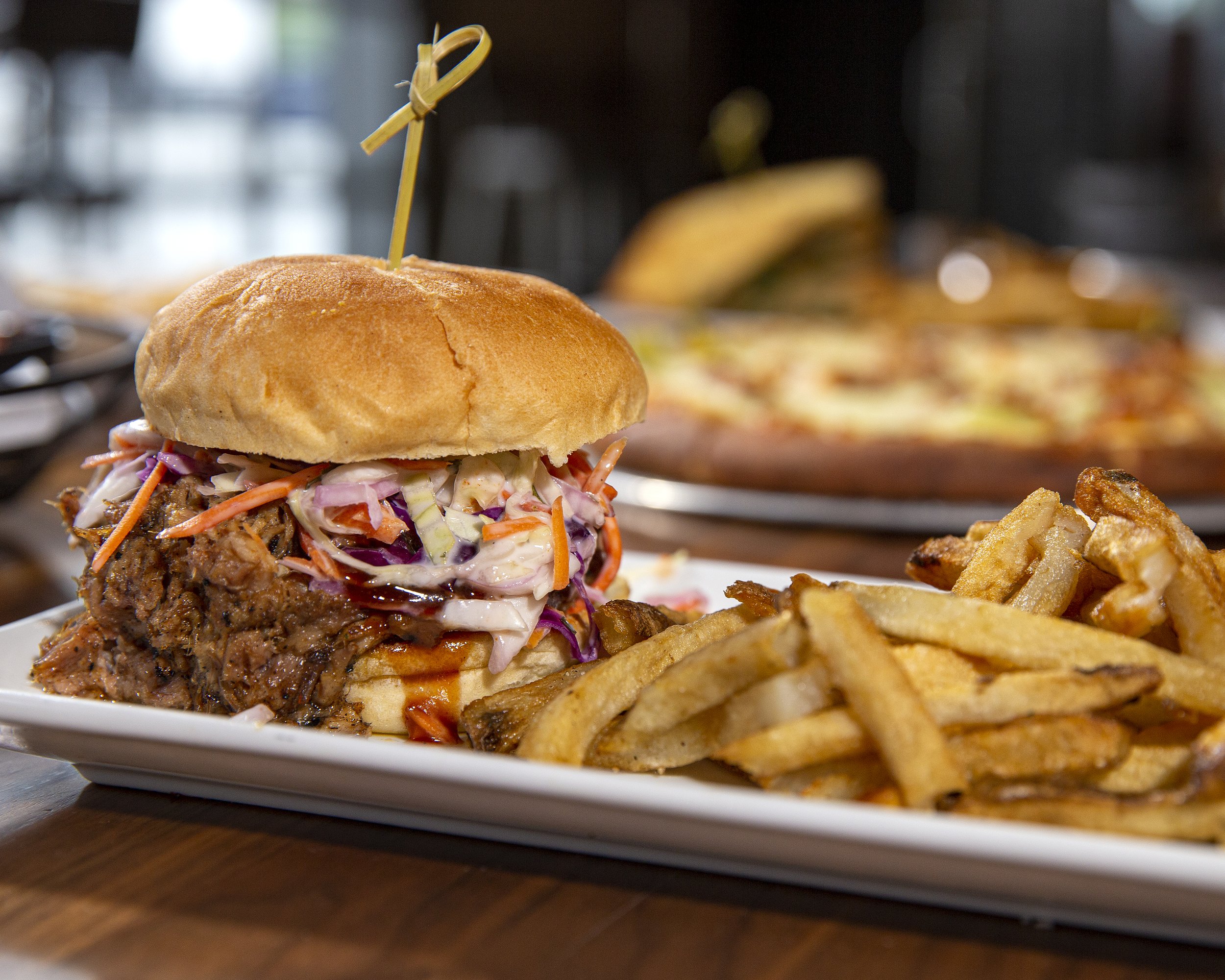This image vividly captures a bustling restaurant atmosphere with a focus on a tempting meal. In the foreground, there's a white rectangular plate presenting a hearty barbecue sandwich and a heap of handmade French fries. The sandwich is assembled with a generous serving of pulled meat, slathered in barbecue sauce and topped with colorful coleslaw made of purple and green cabbage along with carrots. A bamboo toothpick with an intricate curly Q design is used to hold the substantial sandwich together. The fries next to it are crispy and golden. Behind this main dish, there are a couple of out-of-focus plates, one that could be a pizza and another, barely discernible, potentially an open-faced sandwich, indicating a lineup of meals ready to be served. The setting features a tabletop that resembles dark-stained wood, contributing to the warm, inviting ambiance of the restaurant.